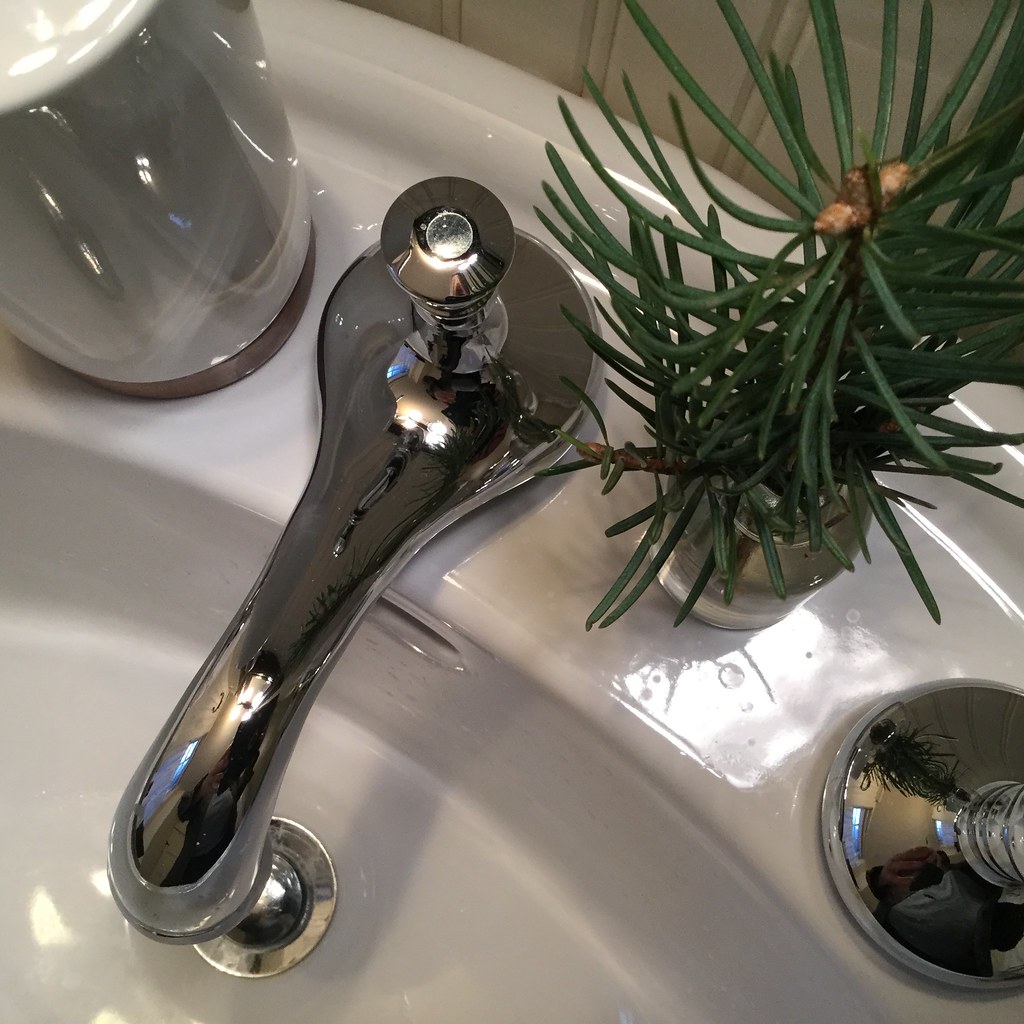This image captures a very close-up view of a white porcelain bathroom sink with a highly polished stainless steel faucet at its center. The reflective surface of the faucet vividly showcases reflections, including light from above, the surrounding plant, and even a hint of the photographer. To the left of the faucet, there's a white ceramic canister partially cut off by the frame. A small houseplant with thin, dark green leaves sits in a clear glass filled with water, positioned to the left, exhibiting a few water droplets around it. The sink features a silver stopper, and we catch a glimpse of a jar with a dark brown base and silver top. The background reveals a stylish wall with thin, cream-colored paneling complemented by beige wood trim.